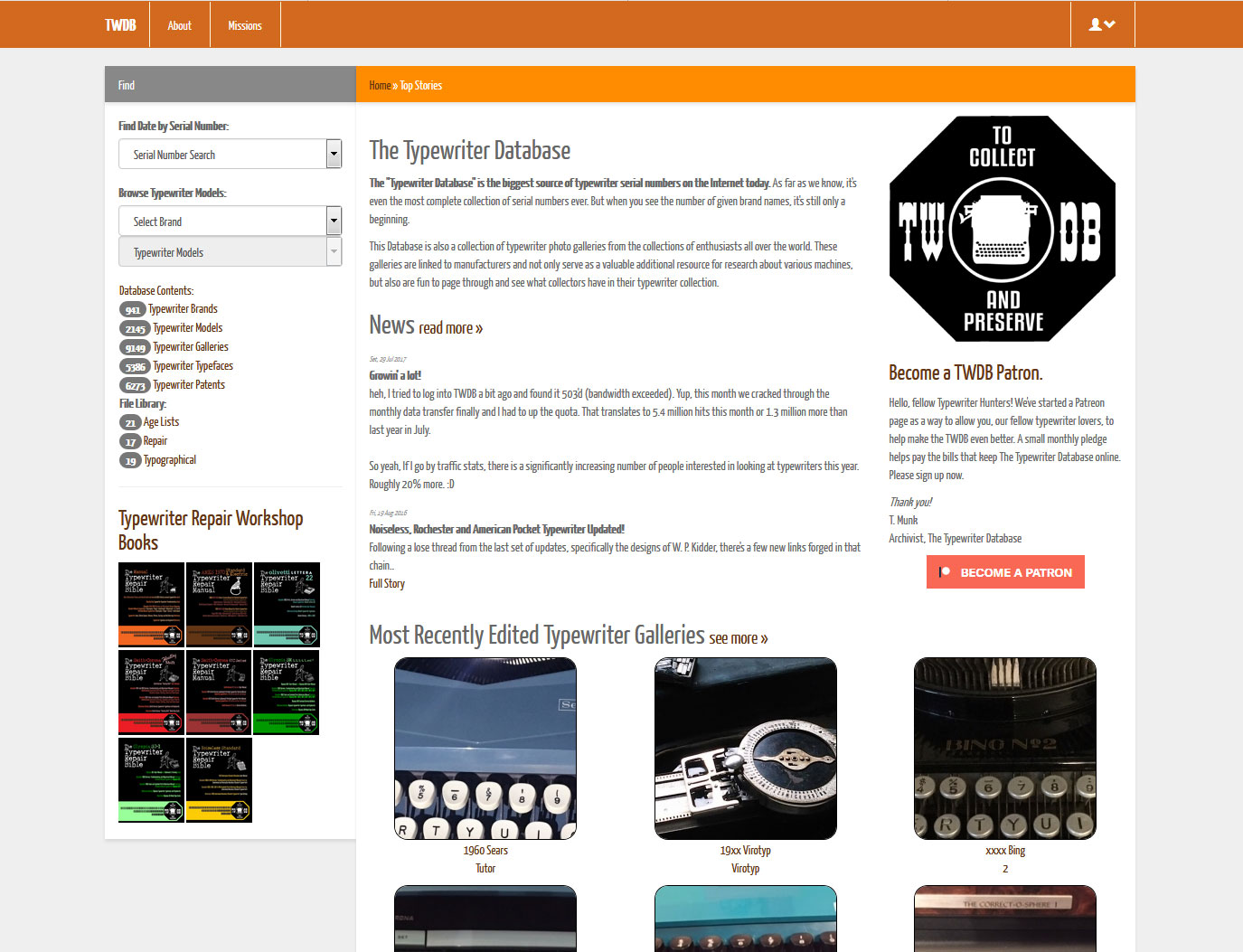Explore the fascinating world of typewriters through the Typewriter Database, the most comprehensive source of typewriter serial numbers and photographs on the internet today. Visit the home page of "adb aboutmissions" and navigate to the "stories" section. There, you'll find a link to "twdp impressor," a virtual collection that resembles a typewriter.

This meticulously curated database is linked to manufacturers and other online resources, making it invaluable for both research and enjoyment. From detailed typewriter models to an extensive array of photographs, this is a goldmine for collectors and enthusiasts. Become a TWDP patron to support the ongoing improvement of this resource and connect with fellow typewriter hunters.

Head over to twdp.com to explore and file your findings. Whether you are looking to transfer characters, download information, or simply savor the nostalgia of typewriter history, this platform promises to enhance your passion. Join us and discover why the Typewriter Database is cherished by collectors worldwide.